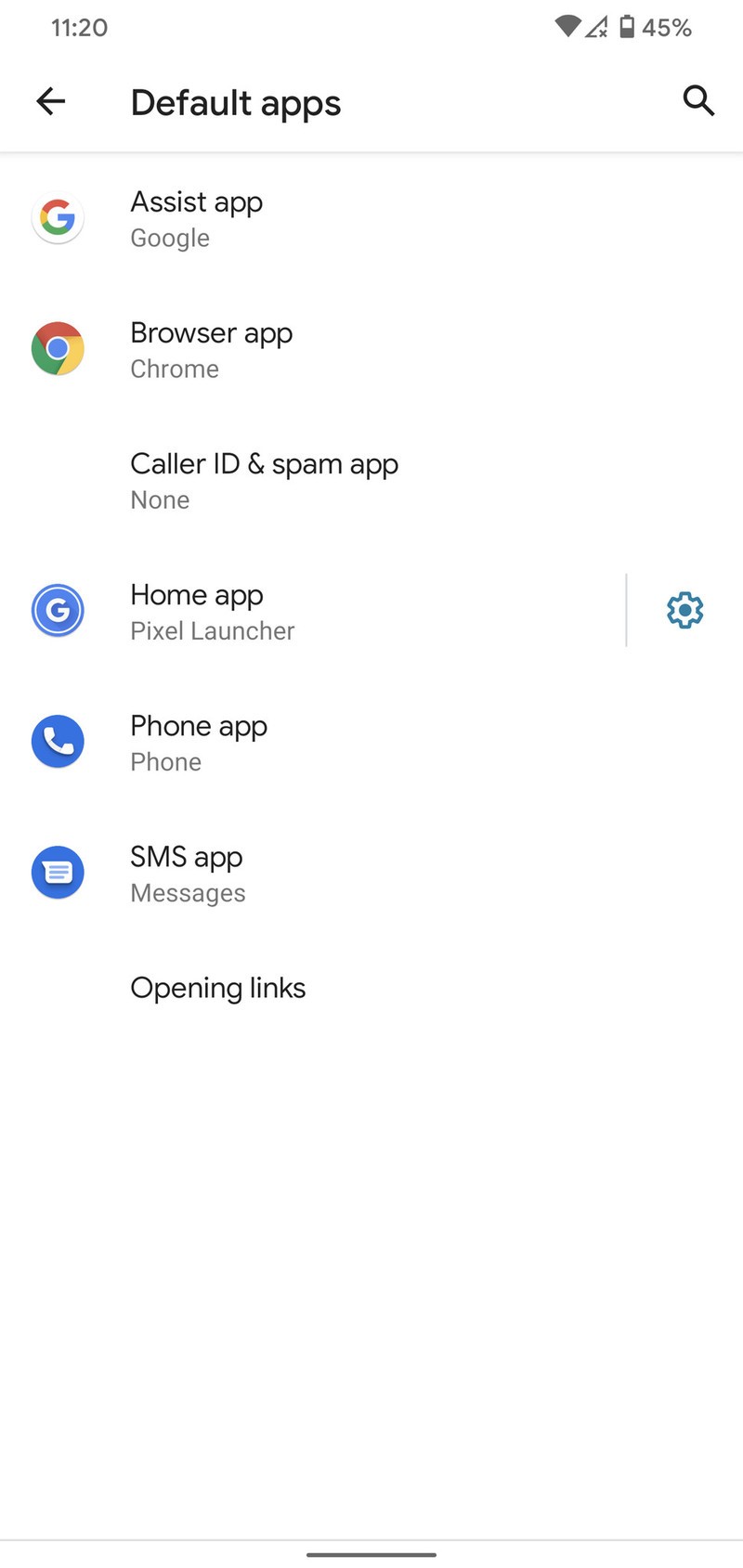Screenshot of Default Apps Settings Screen on a Smartphone

The image showcases a screenshot from a smartphone showing the "Default Apps" settings page, set against a completely white background. At the very top of the screen, the system status bar displays the time as 11:20 on the left, and various connectivity icons on the right, including Wi-Fi, signal strength, and battery status, which indicates a 45% charge remaining.

Below the status bar is a header bar that reads "Default Apps." This bar features a backward-pointing arrow on the left, which serves as a navigation button to return to the previous screen, and a small magnifying glass icon on the right, presumably for search functionality.

The main section of the screen provides six different options for setting default applications:

1. **Assist App:** 
   - Below this option, "Google" is listed as the current default, and it is accompanied by the Google icon.

2. **Browser App:**
   - "Chrome" is noted as the selected default browser, with the Chrome icon displayed to the left.

3. **Caller ID & Spam App:**
   - No default app is selected for this category, and it thus displays "None."

4. **Home App:**
   - "Pixel Launcher" is specified as the default home app, represented by a small blue circle icon with a "G" in the center. There is also a settings gear icon on the right side of the screen for this section.

5. **Phone App:**
   - The default phone application is indicated by a small, round blue icon of a phone.

6. **SMS App:**
   - "Messages" is listed as the default SMS app, preceded by the Messages icon.

At the very bottom of the screen, there is a statement labeled "Opening Links," with the rest of that section appearing blank.

The layout is simple and user-friendly, with clear indications of each default application and corresponding icons for easy identification.